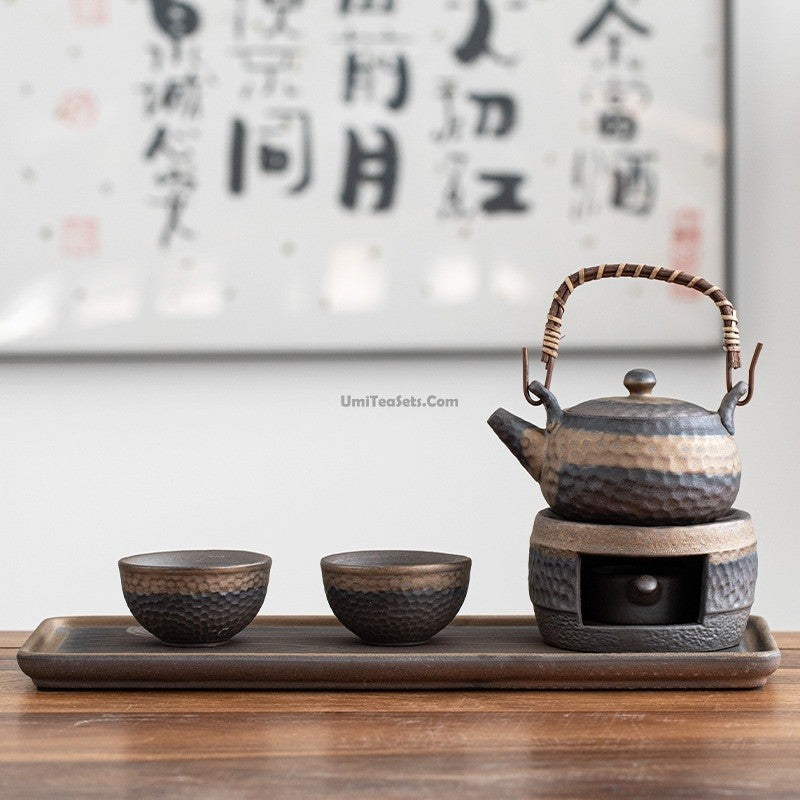Set against a crisp white background, this detailed photograph features a stylish tea set artfully arranged on a brown wood grain table. Dominating the background is a framed piece of calligraphy adorned with large Chinese characters arranged in five rows, adding an element of cultural elegance. This background image is slightly blurred, bringing the focus sharply onto the tea set in the foreground. The tea set consists of a hammered metal tray on the left, holding two textured cups that feature a dark charcoal base with a bronze-colored rim. To the right, a matching tea kettle—with a dark bronze bottom and top, and a bronze center—sits atop a cylindrical stand. The kettle is accentuated by a wooden handle wound with straw, harmonizing beautifully with the cups. An inscription reading "umitesets.com" is prominently displayed in the foreground, centering the viewer's attention on this sophisticated arrangement.